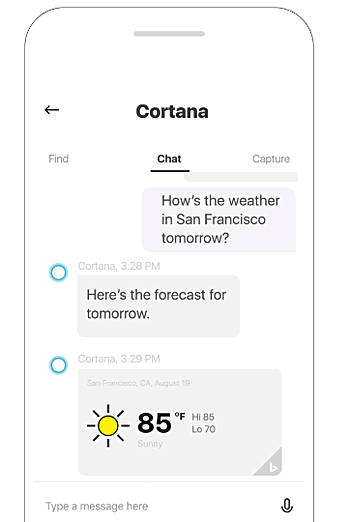In this detailed image, we observe a smartphone screen showcasing a chat interface, likely from an iPhone or an Android device. At the top of the screen, the header displays "Cortana" with a back button positioned to the left. Below this header, there is a navigation menu highlighting three tabs: "Find," "Chat," and "Capture," with "Chat" currently active.

In the chat window, a user query reads, "How's the weather in San Francisco tomorrow?" at 3:28 p.m. Cortana, the AI assistant, responds promptly, providing the weather forecast. The first response at 3:28 p.m. states, "Here's the forecast for tomorrow," followed by a second message at 3:29 p.m. that details: "San Francisco, California, August 19th," accompanied by a sunny icon and temperature details indicating a high of 85°F and a low of 70°F.

Beneath the chat bubble, there is an input section that allows the user to type a message to Cortana. Additionally, a microphone button is available, enabling voice input for hands-free interaction. The entire interface features a clean, minimalist design with a white background and gray text boxes, providing a straightforward layout for ease of use. This image effectively demonstrates the functionality and user interface of the Cortana AI assistant application on a smartphone.